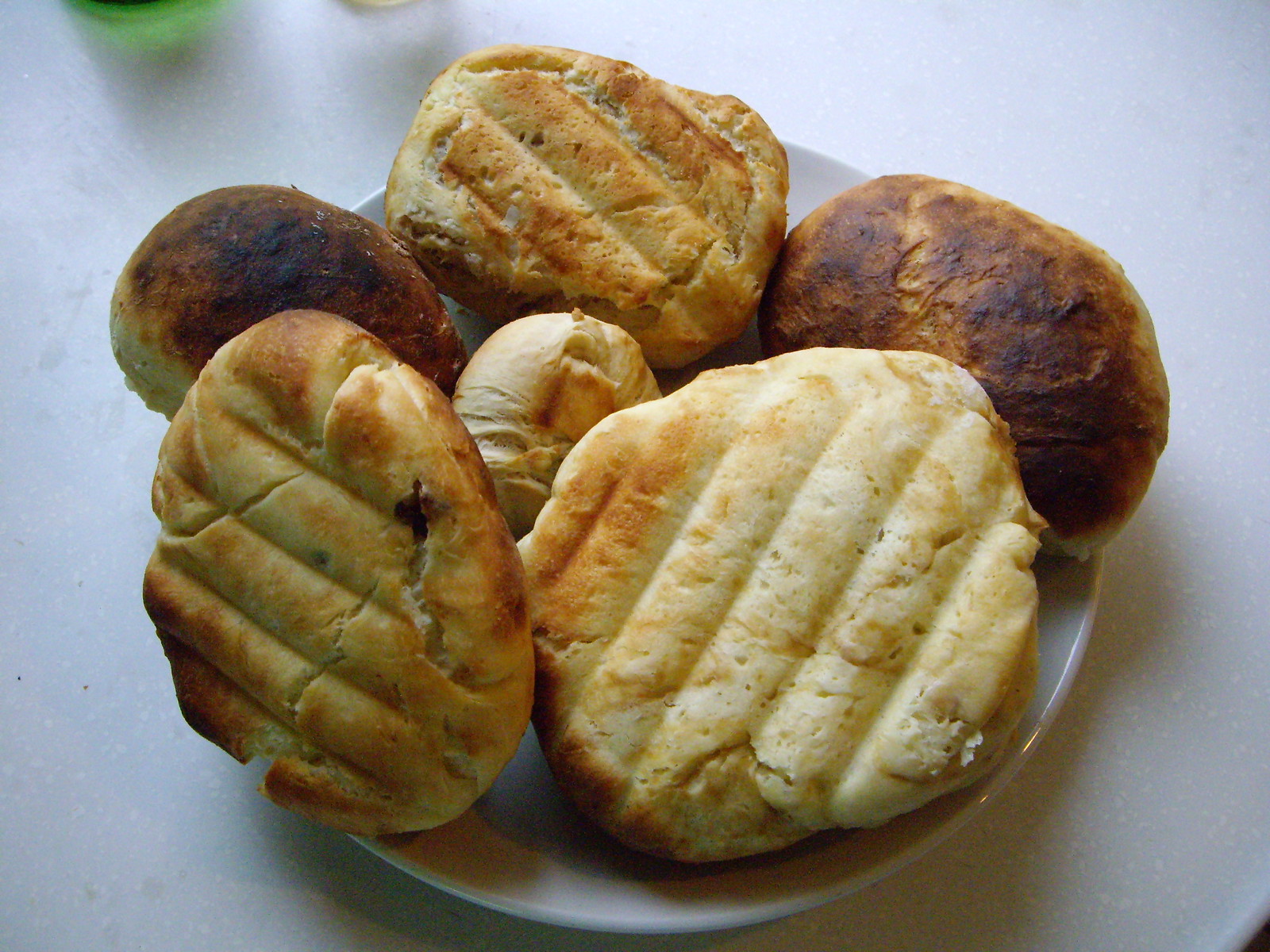This is a detailed photograph showcasing a small, round, white plate made of a reflective material, likely porcelain, ceramic, or china, placed on a white kitchen countertop. The plate is filled to near capacity with six homemade rolls of varying sizes and colors. Some are golden brown while others are deep brown, indicating different levels of baking. The rolls exhibit grill marks, suggesting they were placed directly on an oven rack during baking. Among them, the one in the middle is the smallest and round. The rolls show signs of possible seasoning with herbs and have a shiny sheen on their surface. In the background, towards the upper left side of the dimly lit and low-grain photograph, there are blurry kitchen items, including a green and a reddish object, likely glass.